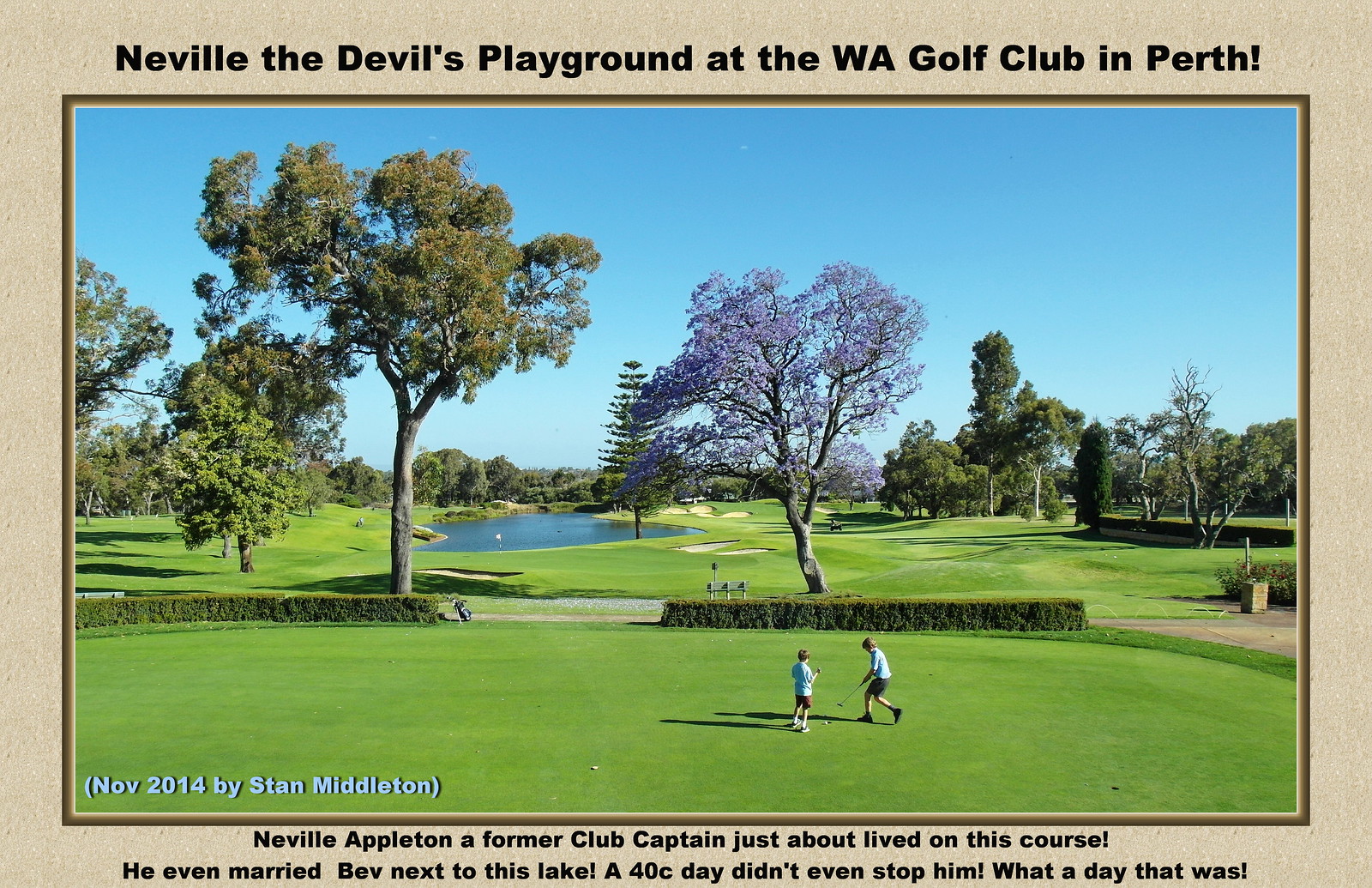The image is a landscape-oriented poster primarily showcasing a photograph of a sunlit golf course at the WA Golf Club in Perth, titled "Neville the Devil's Playground" in black text on a brown background at the top. The foreground of the photograph features a pristine putting green with manicured grass, where two children, both dressed in blue t-shirts, shorts, and trainers, are playing golf. One child is poised with a golf club, ready to putt a ball. Surrounding the green are diverse trees, including both coniferous and deciduous varieties, as well as some flowering bushes. In the background, you can see a lake, sand traps, and possibly a pin. The sky is clear blue, and the entire scene is bathed in bright sunshine. At the bottom left-hand corner of the picture, there is a note in brackets that reads, "November 2014 by Stan Middleton." Beneath the photograph, additional text states, "Neville Appleton, a former club captain, just about lived on this course. He even married Bev next to this lake. A 40C day didn't even stop him. What a day that was."